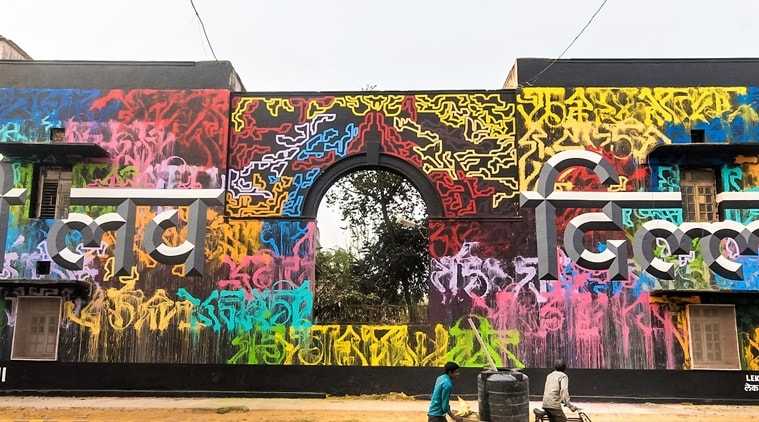The image depicts an urban scene featuring a large, black, industrial-looking building complex that stands two to three stories tall. The buildings are heavily covered in vivid graffiti, with colors including yellow, white, blue, red, pink, orange, and brown. These colorful graffiti artworks cover the buildings' surfaces, giving off a chaotic and messy vibe. Some of the graffiti appears as melting pink letters, and there are areas of raised, silver text that have a futuristic look.

In the center of the buildings, there's an arched walkway or window, also adorned with graffiti. Behind the archway, you can see trees, suggesting a natural backdrop. Above the buildings, the sky is overcast and white, intersected by multiple power lines with cables visible stretching across the scene.

In the foreground, there's a dirt road and a black bin. Two men, one in a gray shirt and the other in blue, are moving near the bin; they appear to be either walking or riding bicycles. Another person in a green shirt is also present in the scene. The overall ambiance is that of a gritty, graffiti-filled urban environment with an industrial and slightly dystopian appearance.